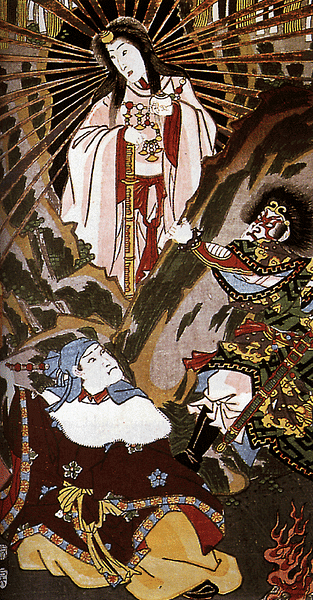This stylized Japanese artwork, possibly dating back around 200 years, vividly depicts a floating female warrior framed by worn, rusty rays that emanate like splintered wood from behind her head. Adorned in a white and pink robe with a red interior, a red belt, a gold ornamental headpiece, and a multicolored necklace, she exudes an imperial aura. Clasping a golden sword at her belt, she looks downward towards a kneeling Japanese man below, dressed in a brown uniform with a yellow bottom and a blue head wrap, seemingly seeking her protection or guidance. To the right, an ominous figure with a painted face and ornate robe, bearing a frightening expression, appears to be restraining or challenging the warrior, adding tension to this dramatic scene.